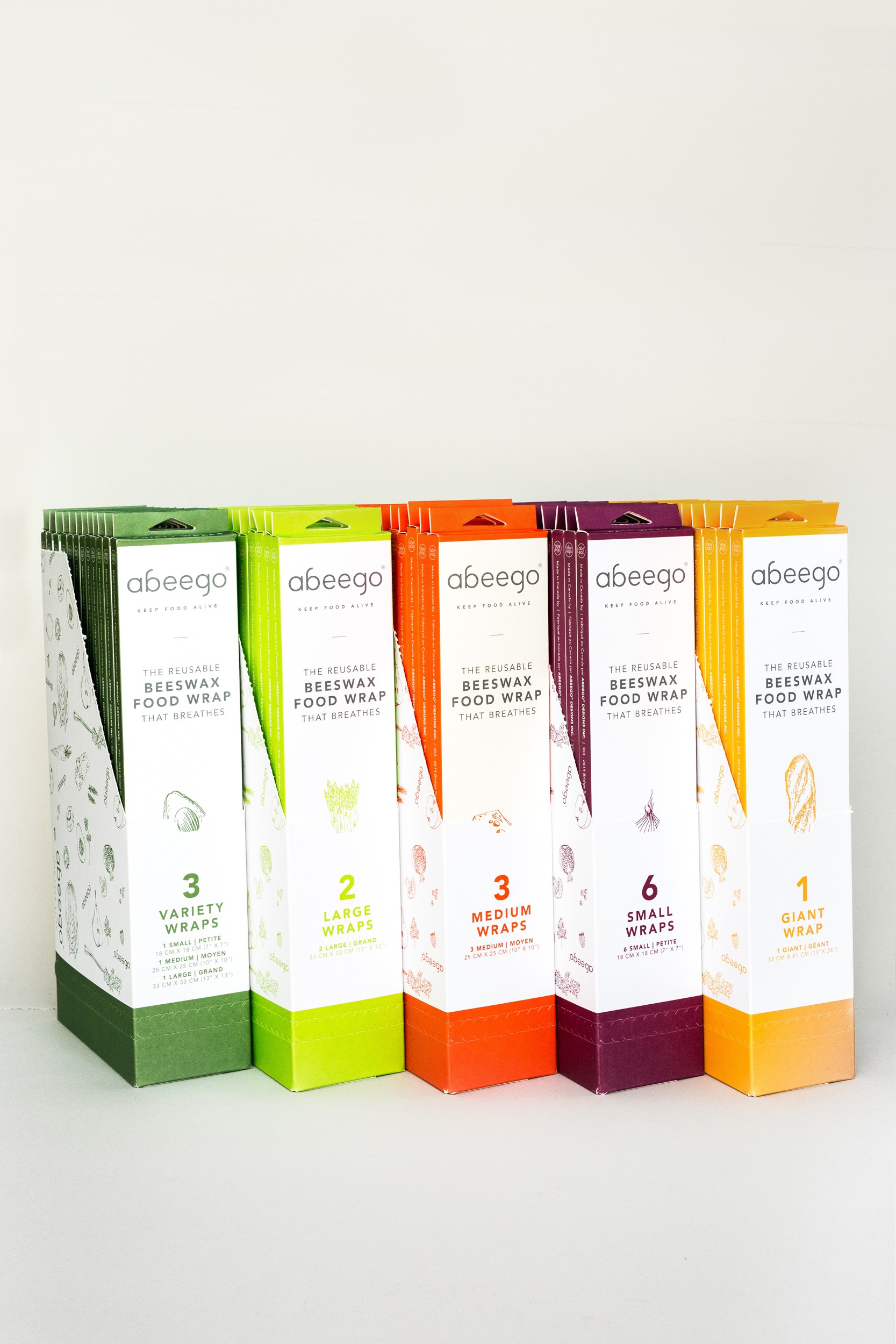This image showcases an assortment of five Abego beeswax food wrap packages arranged side by side in an indoor setting. Each package is a different color and size variation, all uniformly branded with "Abego" in black letters on a white background, and the phrase "Beeswax Food Wrap" prominently displayed. 

Starting from the left:
1. A green package with images of food items and a sleeve that reads "three variety wraps".
2. A yellow package labeled "two large wraps".
3. An orange package marked "three medium wraps".
4. A purple package indicating "six small wraps".
5. Another yellow package featuring an orange band and stating "one giant wrap".

The background of the image is a neutral gray, highlighting the vibrant colors of the packaging and emphasizing the variety and utility of the Abego beeswax food wraps.